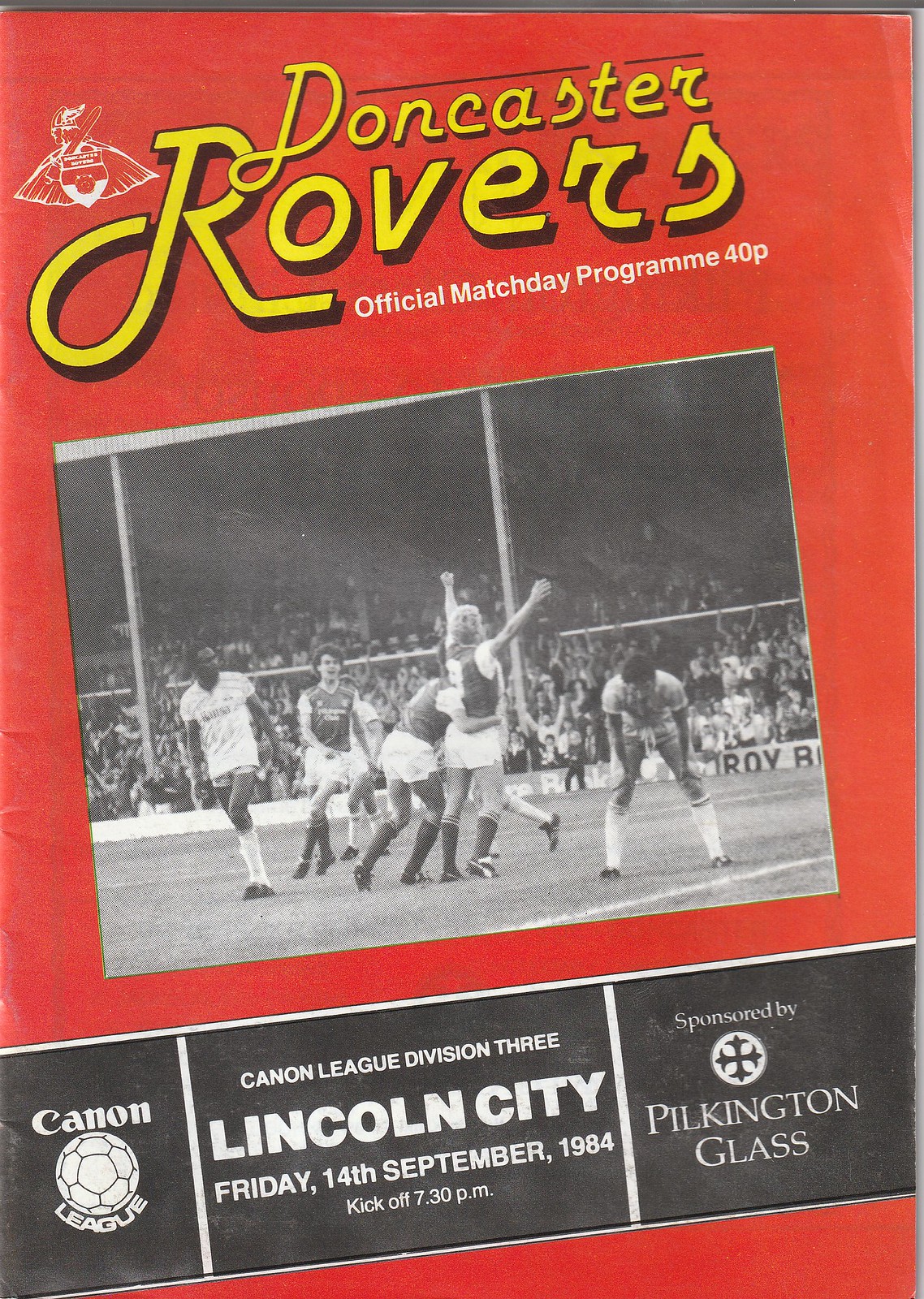The image is the cover of a match day program for a European soccer event, featuring the Doncaster Rovers. The background is deep red with "Doncaster Rovers" prominently displayed in bold yellow text at the top. Just below, the text reads "Official Match Day Program 40p" in white. The top left corner showcases the club’s crest, depicting a figure with a sword. 

Dominating the center of the cover is a black and white photograph capturing a group of multi-ethnicity players in celebration, likely after a goal. The scene is set against the backdrop of a packed stadium with enthusiastic fans cheering in the stands. 

At the bottom of the cover, a black-and-white banner provides more details: on the left, it features "Cannon League" accompanied by a soccer ball icon; in the center, it lists the match specifics: "Division 3, Lincoln City, Friday 14th September 1984, kickoff 7.30pm"; and on the right, it notes the sponsorship by "Pilkington Glass" along with its logo.